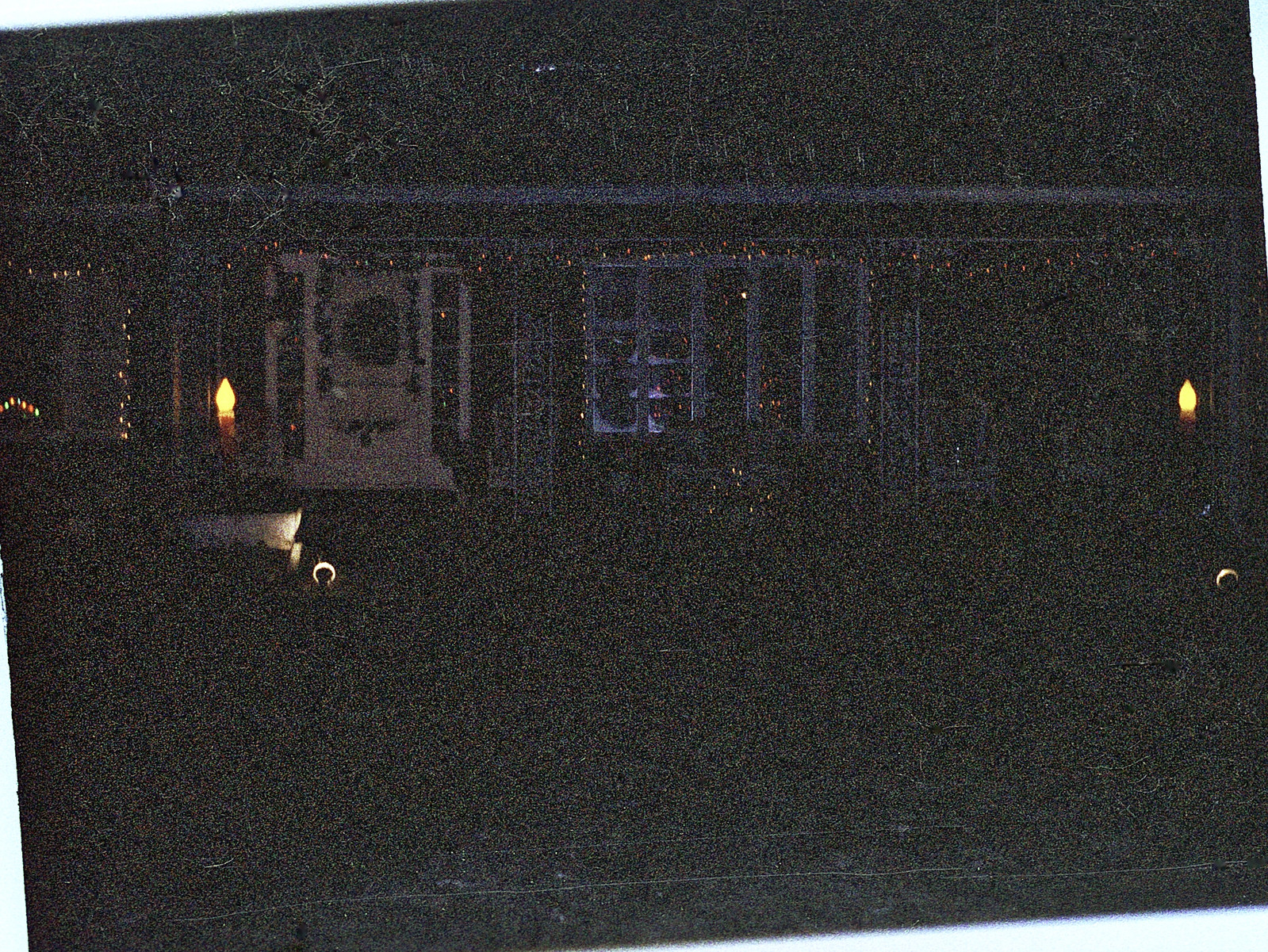The image depicts a highly pixelated and dark photograph of a one-story house, presumably taken from an old, grainy photo. The house is decorated for Christmas, noticeable by the faint outlines of colorful Christmas lights—red, yellow, blue, and green—around the windows and doors. A white door is barely visible, framed by vertical windows on either side, adorned with a possible wreath. The front yard features two candle-like decorations emitting an orange glow, likely plastic seasonal ornaments. The poor quality of the image, with its scratch marks and white static circles, adds to the overall difficulty in discerning finer details but strongly suggests a festive, albeit obscured, holiday scene.